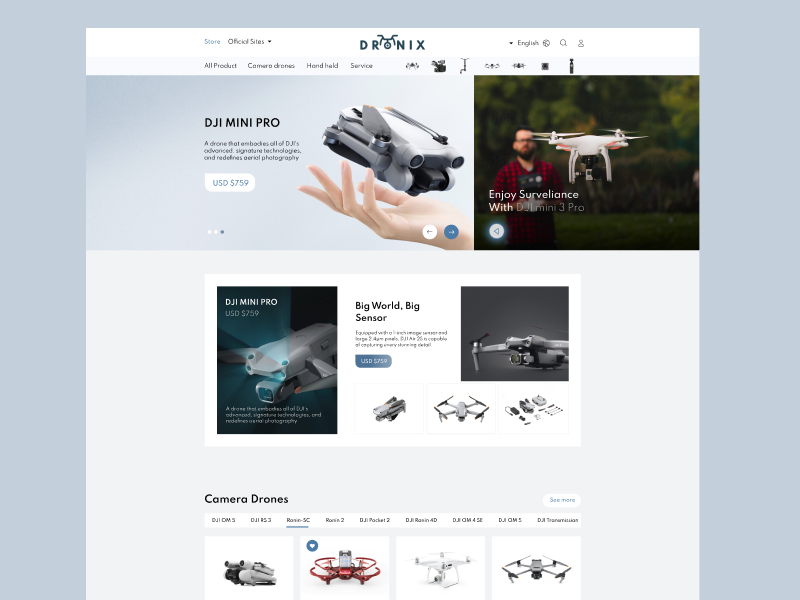The image appears to be a screenshot of a computer screen displaying a webpage. The background is gray, with a prominent white rectangular section in the center. At the top of this white section, there is text that reads "Official Site," accompanied by a drop-down menu option. To the right, in blue, is the stylized text "DRONIX," with a drone icon hovering over the letter "O." Further to the right are options for language selection (set to English), a search icon, and an account icon.

Below this header section, there are navigation options reading "All Products," "Camera Drones," and "Handheld Service." Directly beneath, two images are displayed side by side. The first image on the left features a gray background with the text "DJI Mini Pro." In this image, a gray drone is shown above an outstretched hand, accompanied by a price tag of "$759."

The second image to the right shows a man outdoors flying a white drone, with the caption "Enjoy Surveillance With DJI 3 Pro." Below this, a rectangular section features an additional image of a drone, labeled "DJI Mini Pro." To the right of this image, text reads "Big World, Big Sensor." This area highlights the compact form, separate parts, and included accessories of the featured drone.

At the very bottom of the white section are four smaller squares, representing the available camera drone options.